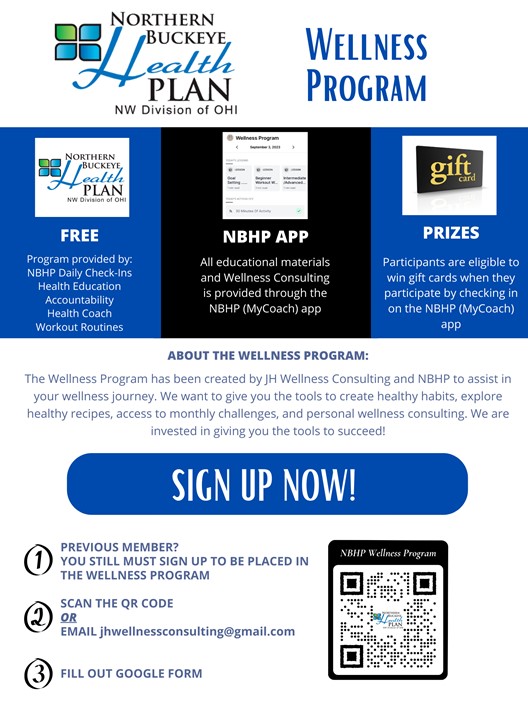This digitally generated poster for the Northern Buckeye Health Plan prominently features the name "Northern Buckeye Plan" in a black font at the top-left corner. Directly beneath it, the subheading "NW Division of OHI" is also in black. Contrasting this, the word "Health" is rendered in a vibrant blue font, matching the blue "Wellness Program" text positioned to the right of the main title. 

The poster's background is predominantly white, accented with various sections featuring black and blue backgrounds. Below the name, a horizontal banner splits into three distinct boxes: the two outer boxes are blue with white text, while the center box is black with white text. These boxes highlight the key features of the wellness program.

Underneath the banner, a detailed blurb describes the wellness program in white font against a black background. Below this blurb, there's a prominent blue button labeled "Sign Up Now" in white font.

Towards the bottom, three steps are clearly delineated with numerals "1, 2, 3" in black font, providing straightforward instructions. Adjacent to these steps on the right side, a QR code invites users to scan and access a Google form for further engagement with the program.